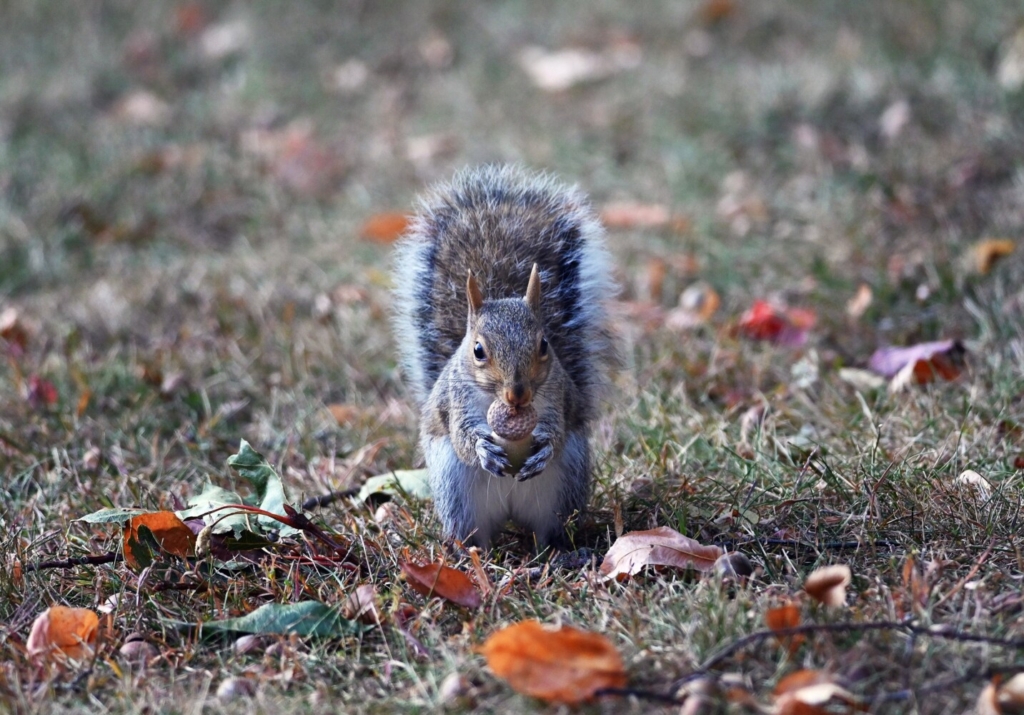Captured in the bright light of an autumn day, this detailed photograph features a brown squirrel with perked-up ears and a bushy tail almost as wide as its body. The squirrel, standing on the ground amidst greenish grass interspersed with crinkly, autumn-colored leaves in hues of orange, red, yellow, and some remaining green, is the central focus of the image. With its tiny paws cupping a large acorn, the squirrel looks directly at the camera, seemingly aware of the photographer's presence. Tiny twigs and branches are scattered around, framing the scene. The clearness of the foreground, where the squirrel's white, black, brown, and gray fur stands out, contrasts with the progressively blurry background, enhancing the squirrel's prominence in this vibrant autumn setting.